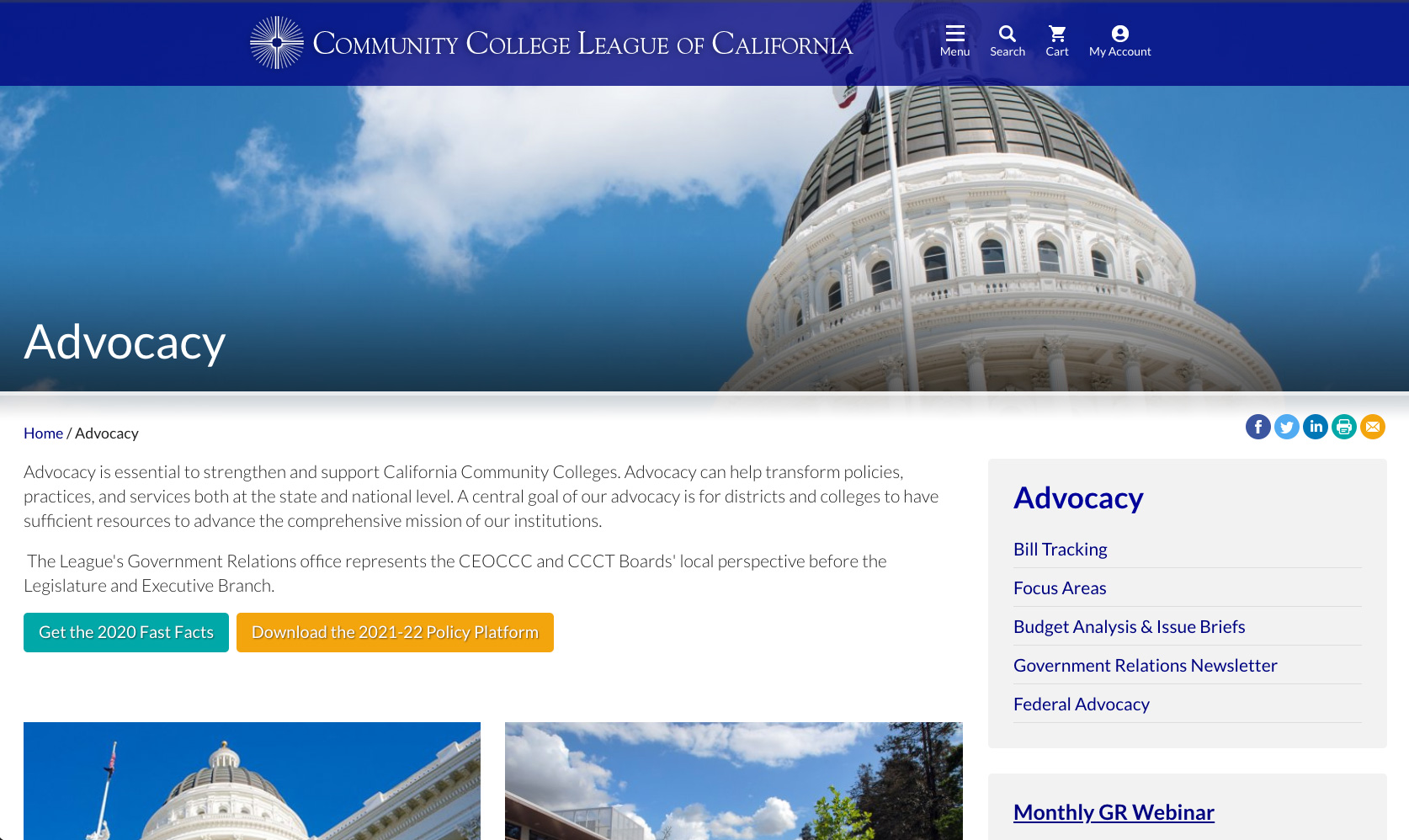The image is a screenshot of a website with a layout that is approximately 50% wider than it is tall. At the very top, occupying about 15% of the image's height, is a dark blue banner featuring the logo of the Community College League of California. The logo consists of a white cross within a circle, followed by the organization's name in text. To the right of the logo, there are four icons labeled Menu, Search, Cart, and My Account.

Below this banner is the main header image, depicting the spire of a building extending into a partly cloudy sky. In the lower left corner of this image, the word "Advocacy" is written in white text.

The next section, covering about one-third of the image's height, has a white background. In the upper left corner, navigation breadcrumbs read "Home / Advocacy." This section contains a couple of paragraphs discussing advocacy, presumably in relation to the Community College League of California. 

On the lower left of this section, there is a teal button labeled "Get the 2020 Fast Facts," and to its right, an orange button labeled "Download the 21 to 22 Policy Platform."

Beneath this are two images that are obscured but seem to depict a spire and possibly another building. In the lower right corner, there is a gray box with dark blue text, which appears to serve as a navigation aid.